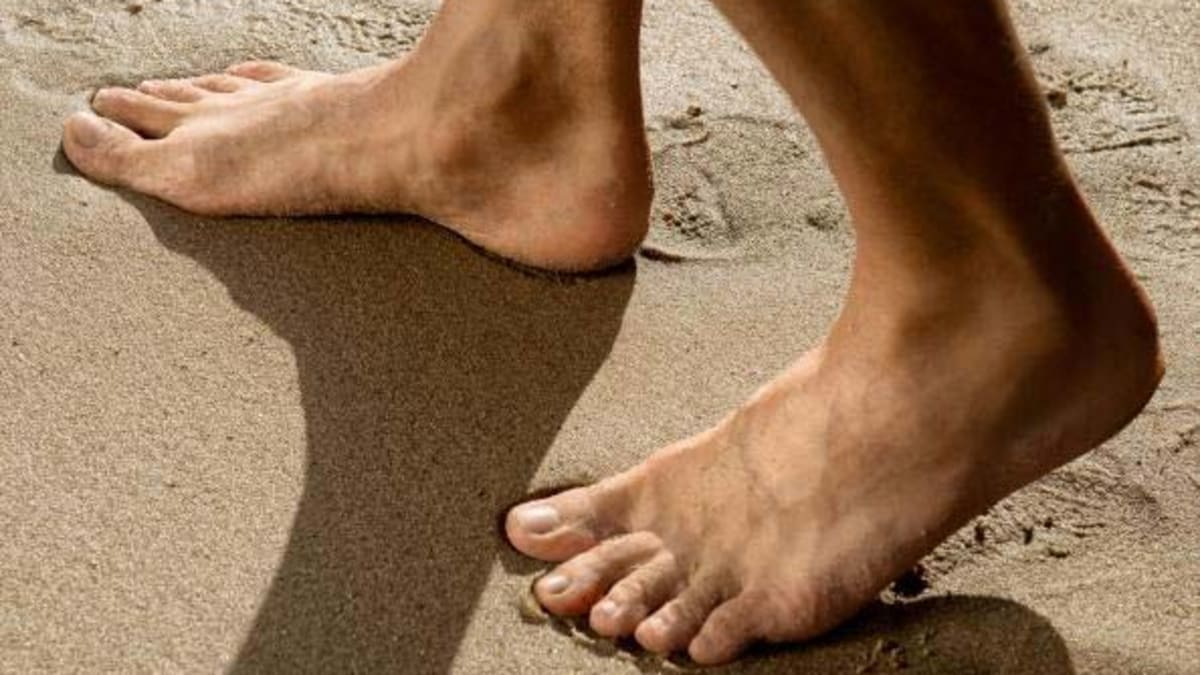The image depicts a person's bare feet walking on wet, dark brown sand, which appears waterlogged and slightly compacted. The feet are shown from the ankles down, with fair skin and well-manicured toenails. The right foot is planted fully on the ground while the left heel is raised, causing the toes to dig into the sand and leaving visible footprints. The sand has a choppy texture from the dampness and is marked with several foot impressions. Both feet cast clear shadows, indicating bright sunlight that also reflects off the sand, enhancing the scene's detail and clarity.